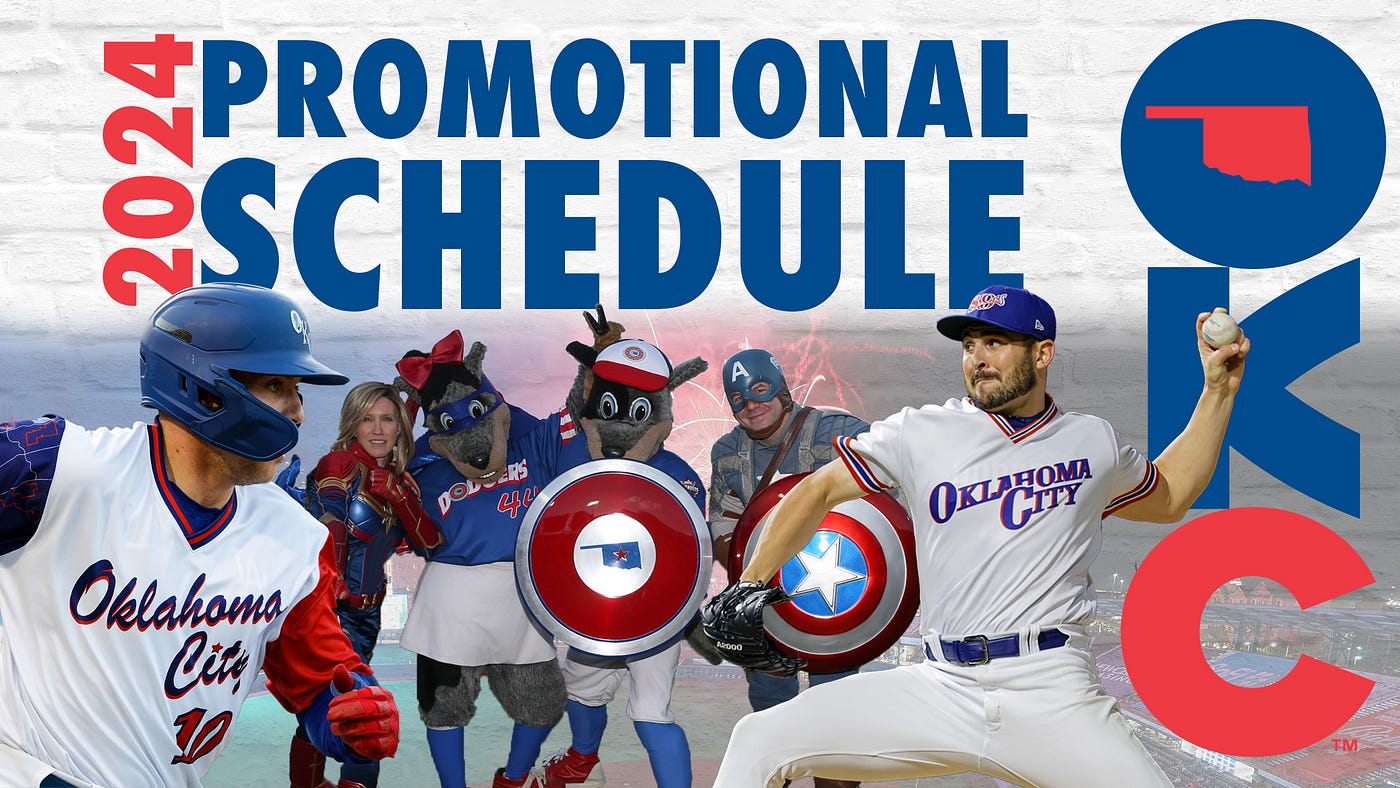In this vibrant promotional poster for the Oklahoma City baseball team's 2024 season, the centerpiece features a pitcher in an Oklahoma City jersey, positioning to throw a ball with his left hand. Flanking him is a variety of captivating characters, all looking towards the center. To the left stands a man dressed as Captain America, brandishing an iconic American shield. Beside him are two mascots—one male with an Oklahoma shield clad in team colors, and a female adorned in a white blouse under a team t-shirt.

Further left, a character dressed as Captain Marvel smiles brightly at the camera. On the extreme left is a baseball runner, seemingly mid-action, hinting at the dynamism of the sport. Dominating the top of the image are the prominent red and blue letters announcing the "2024 Promotional Schedule," with "2024" in red text and the words "promotional" and "schedule" arranged vertically in blue. The right side of the design features the bold letters "OKC," where the 'O' encloses a red silhouette of the state of Oklahoma. The combination of spirited mascots, superhero outfits, and an action-ready team encapsulates the excitement of the upcoming season.